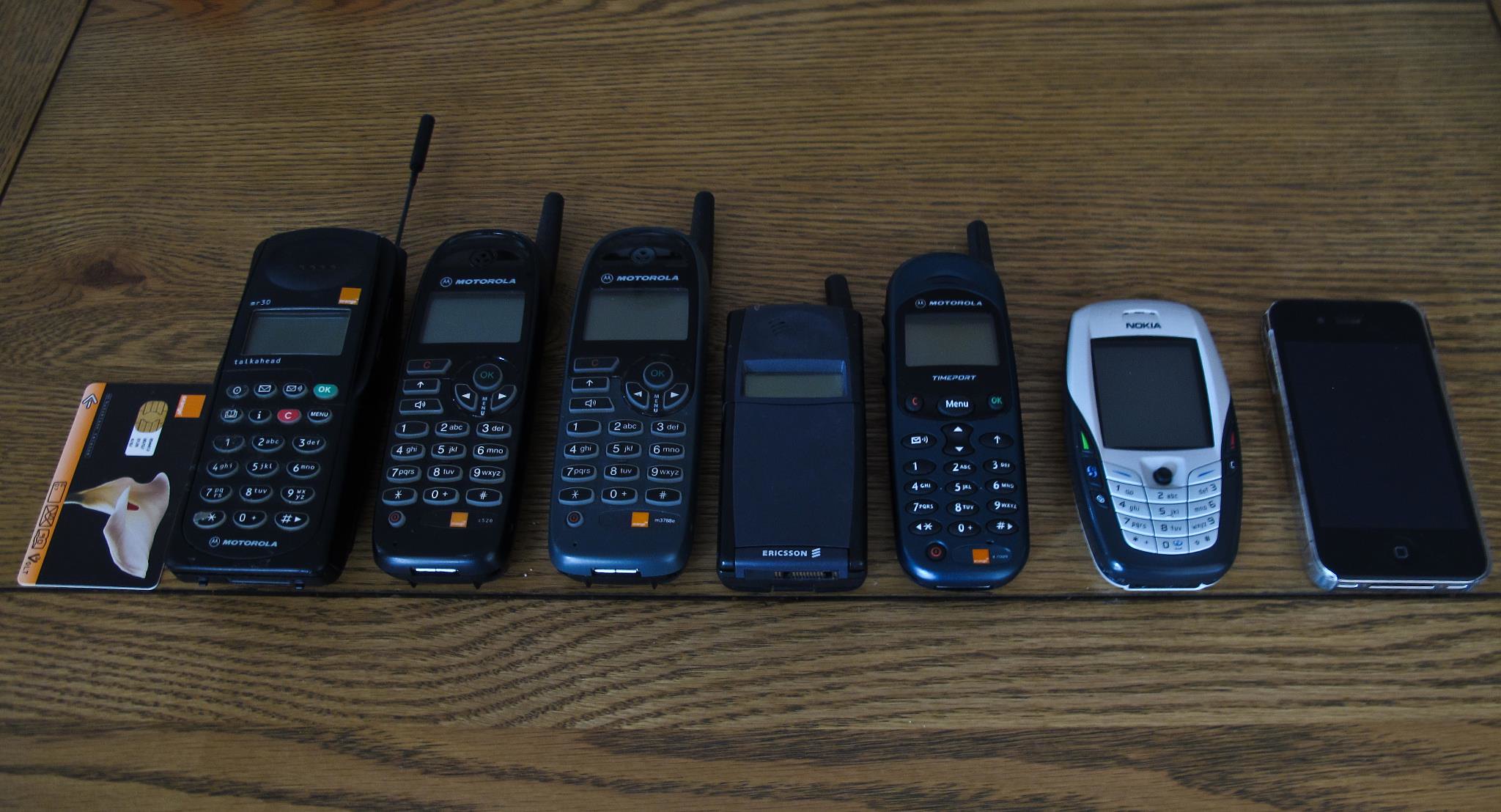This image is a color photograph of seven old cell phones of various models, meticulously laid out side-by-side on a wooden surface, likely a desk. Most of these cell phones, which date back to earlier generations of mobile technology, are black, rugged, and brick-like in appearance, characteristic of older Motorola models. In contrast, one phone is white with black outlines and stands out with a larger screen and white buttons. Notably, the collection includes an array of designs, from a thin, credit card-like object to early handheld phones with antennas - one with a long, extendable antenna and two with shorter, nubby antennas. Among the lineup is a bluish flip phone, suggesting the evolution of mobile designs over the years. The last device on the right appears to be a more contemporary smartphone, possibly an earlier model iPhone or similar, highlighting the transition in mobile technology. To provide a sense of scale, a card is also placed alongside the phones. The overall arrangement presents a visual timeline of the technological advancements from early handheld devices to modern smartphones.